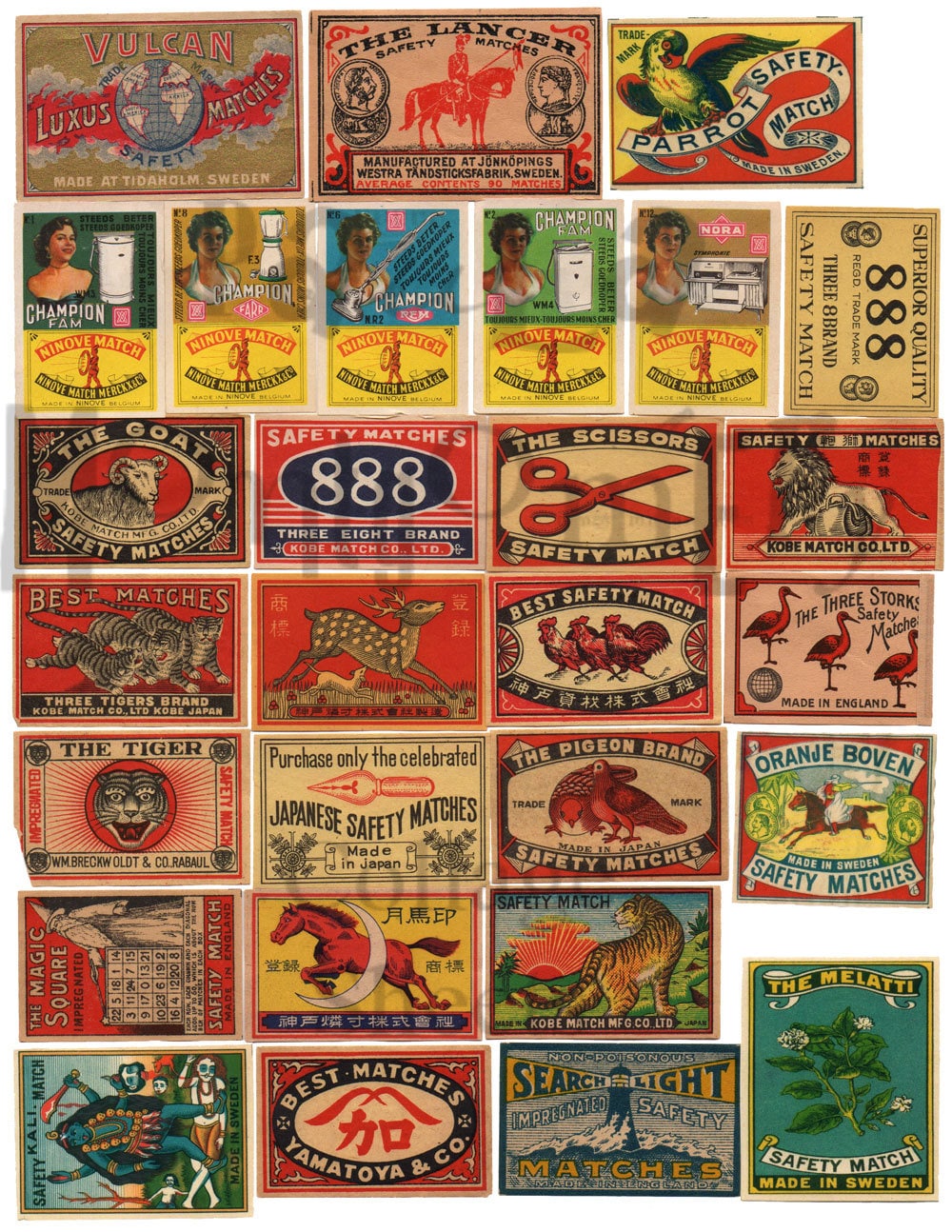This captivating collage consists of a photograph—or possibly a scan—of an array of vintage matchbox covers, meticulously displayed against a pristine white background. The matchbox covers are arranged in a neat grid, with some touching edges while others are separated by small gaps of white space. Each cover showcases a variety of nostalgic and intricate illustrations, including roosters, a serene deer, majestic tigers, an elegant horse, a picturesque lighthouse set against a landscape, a delicate plant, and various birds. Prominently featured is the number "888", suggesting some thematic significance. The matchbox covers primarily adhere to a rectangular shape, though there are notable variations with some being square and others elongated in a vertical orientation. Among the assortment, a series of "Champion" branded covers stands out, distinguished by the portrait of a woman. The color palette is predominantly red and sepia tones, interspersed with subtle hints of yellow, green, and dark blue, evoking a sense of vintage charm and timelessness.